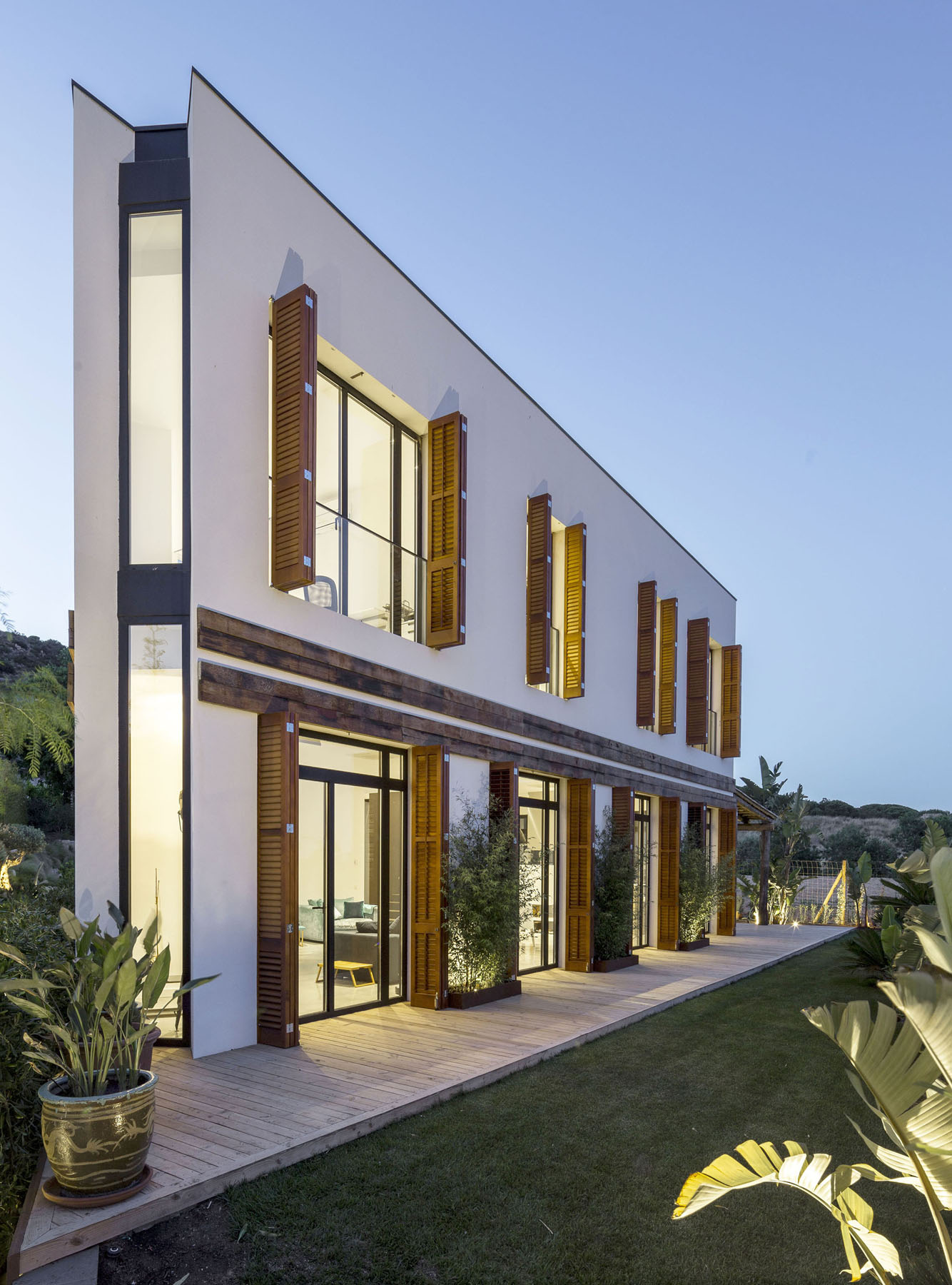The image depicts a uniquely designed, futuristic concept home taken during daytime, possibly in a desert-like area. The two-story structure stands out due to its strikingly narrow, almost triangular form when viewed from an angle. The building’s exterior is primarily white, featuring full-sized glass doors and large rectangular windows with wooden shutters on both floors. A light-gray wooden patio extends from the base, surrounded by well-maintained, neatly trimmed green grass and various plants, including banana and fern-like species. The front face of the building, presenting substantial width, contrasts sharply with its slender side profile, giving the appearance of being almost flat. The sky overhead is a light blue, suggesting it is either early morning or late evening.